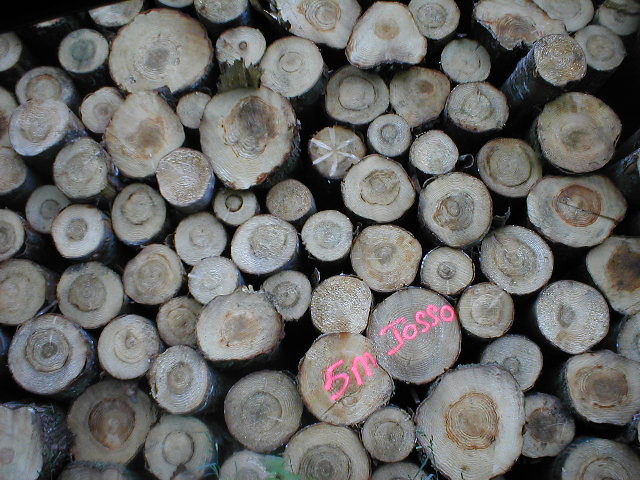This detailed overhead photo showcases a large, varied collection of chopped tree trunks, each displaying their unique tree rings and knots. The trunks, a blend of grays, beiges, darker browns, and rust colors, are closely packed together, resembling stacked firewood. Near the bottom left extending to the mid-right of the image, there is a noticeable pink spray-painted text that reads "5M JOSSO," with the letters spread across multiple logs. Additional interesting details include a faint white starfish-like marking on a tree trunk positioned approximately three rows down from the top, slightly north of the center. The trunks vary in size and shape, with some displaying prominent, large rings while others have barely visible ones, contributing to the overall textured and intricate pattern.